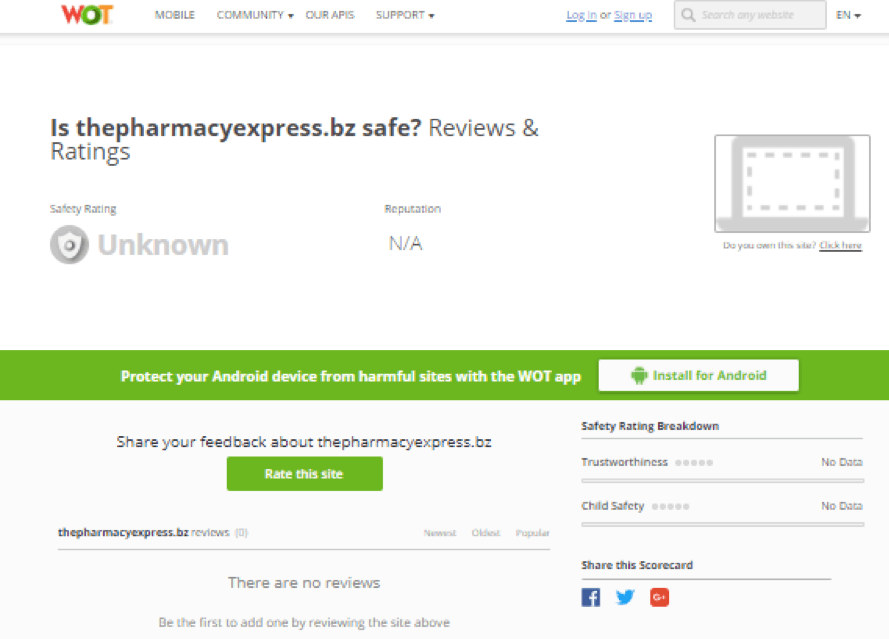The screenshot showcases a web page with a clean, white background. In the top-left corner, there's the word "WHAT," stylized with a red "W," green "O," and orange "T." To the right, in gray text, the navigation options are listed: "MOBILE," "COMMUNITY," "OUR APIs," and "SUPPORT." Adjacent to these, a blue hyperlink labeled "LOGIN" sits alongside another that reads "SIGN UP." A search bar with the placeholder text "SEARCH ANY WEBSITE" is positioned to the far right. A light gray line runs horizontally beneath these elements, spanning the entire width of the page.

Below this line, in bold black letters, the text reads "Is the PharmacyExpress.bz safe? Reviews and ratings." Directly underneath, it states "SAFETY RATING: UNKNOWN," and "REPUTATION: NOT APPLICABLE." A prominent green box below contains the message, "PROTECT YOUR ANDROID DEVICE FROM HARMFUL SITES WITH THE WHAT APP," accompanied by a clickable white rectangular box. This box features a green robot icon and green text that says "INSTALL FOR ANDROID." Further down, there’s an invitation to "SHARE YOUR FEEDBACK ABOUT THE PHARMACYEXPRESS.BZ," followed by a green box with the prompt "RATE THIS SITE."